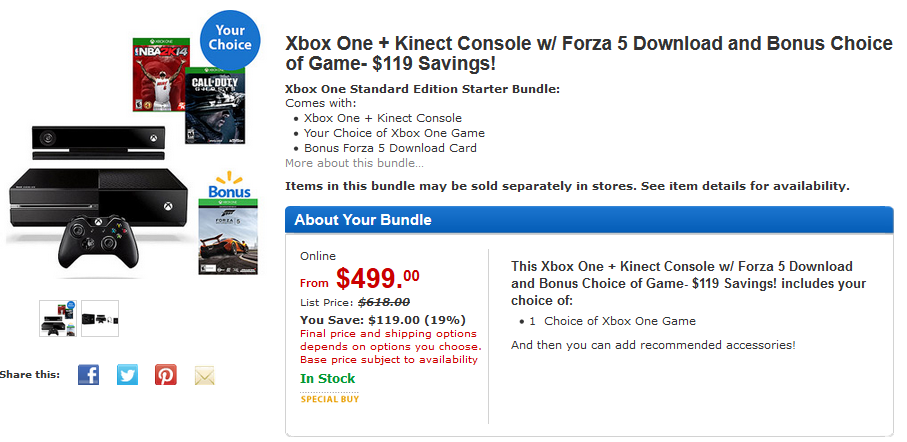This image showcases a detailed web page listing for an Xbox One with Kinect console bundle, featuring promotional savings and various purchasing options. The key highlights of this offer include:

- **Product:** Xbox One with Kinect console
- **Edition:** Standard Edition
- **Bundle:** Tata Bundle
- **Extras:** 
  - Bonus choice of one Xbox One game
  - A five-download card
- **Pricing:**
  - **Initial List Price:** $618
  - **Discounted Online Price:** Starting from $499
  - **Total Savings:** $119
  - **Savings Percentage:** Approximately 19.25%
- **Availability:** Items in this bundle might be sold separately in retail stores, and availability varies. Check item details for more information.
- **Final Price & Shipping:** Final cost and shipping options may depend on additional selections made during the purchase process.
- **Special Buy:** This offer is categorized as a special buy, emphasizing its limited availability or exclusive nature.

This listing provides a comprehensive overview of the bundle, its benefits, and purchase conditions, ensuring customers have all necessary information before making a decision.